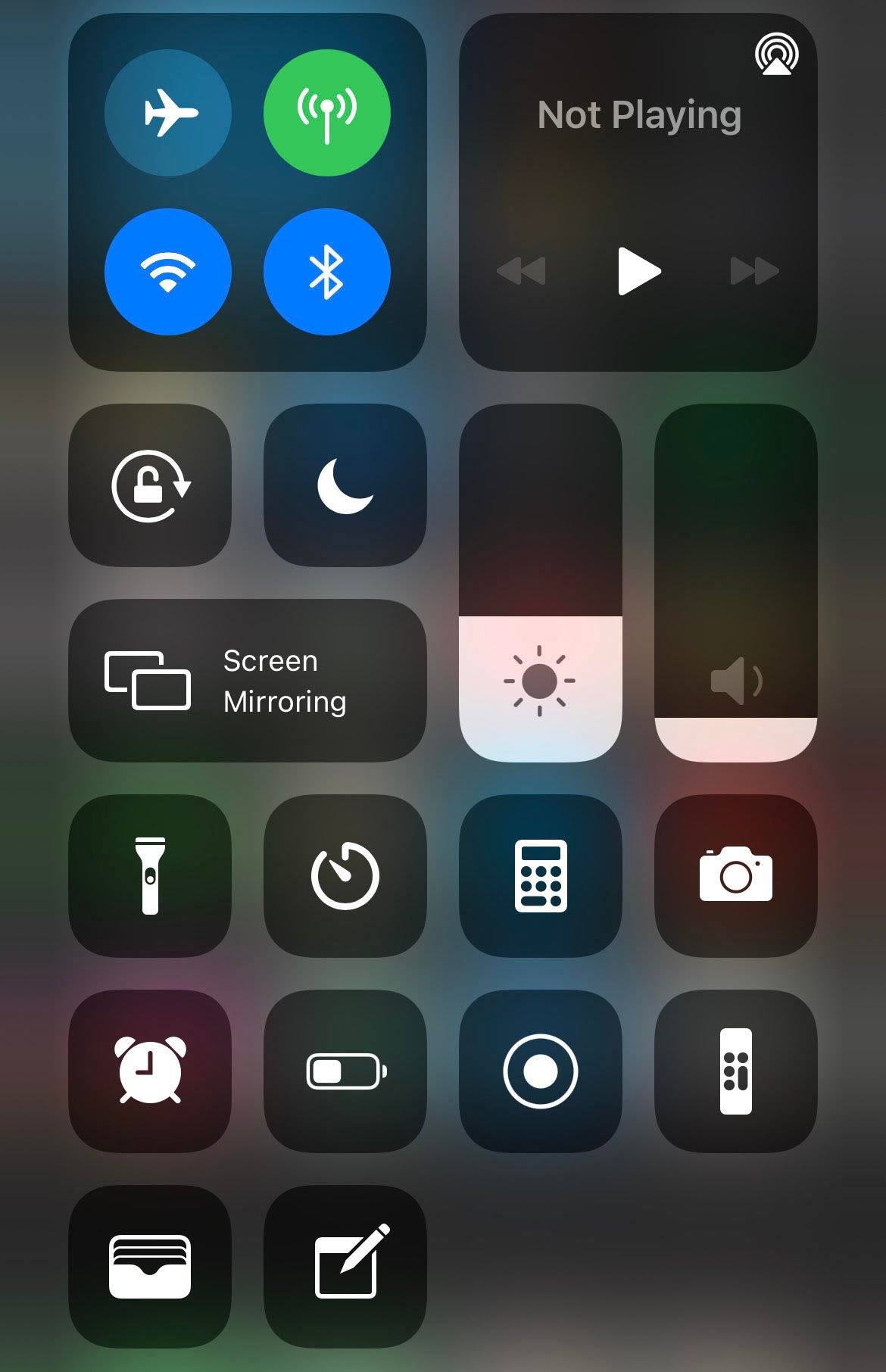This screenshot showcases a smartphone's control center, divided into neatly arranged square and rectangular sections with rounded corners. The top-left square contains toggle options for Airplane Mode, Wi-Fi, Bluetooth, and an unfamiliar network signal icon. Adjacent to it on the right, a square box labeled "Video" indicates a paused state with a play button, flanked by fast-forward and rewind controls. Additional controls include a lock icon in the center of a circle, a circular arrow for screen rotation, a crescent moon for Do Not Disturb mode, and a block labeled "Screen Mirroring." There are also sliders for screen brightness and sound adjustment. Further sections feature icons for a flashlight, calculator, camera, timer, and alarm, along with a battery indicator and several other unrecognized icons.